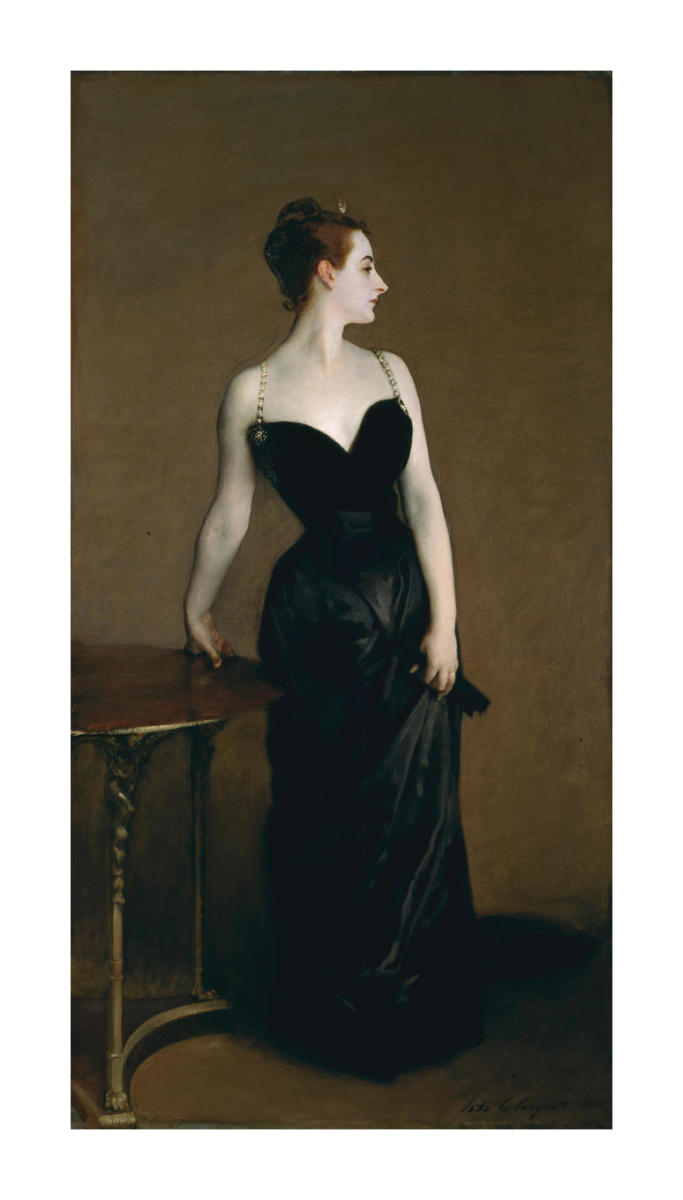The image depicts a realism painting from the early 1900s of a woman in an elegant black evening dress, detailed with gold metal shoulder straps that leave her arms and neck exposed. The woman, portrayed with milky white skin, has her brown hair pulled back into a bun, and her facial features include a distinctive pointy nose as she looks to the left side of the painting. Her pose is graceful yet composed, with her right hand resting on a thin, short wooden table at her side. The lower part of her long, flowy dress reaches the brownish floor, adding to the overall elegance of her appearance. The background features a yellowish-brown hue, with the light source subtly illuminating her from the right, enhancing the lifelike quality of the painting. The intricate detail in her attire and surroundings gives the artwork a photographic realism, capturing the poised beauty of the woman as she possibly readies herself for an evening out.